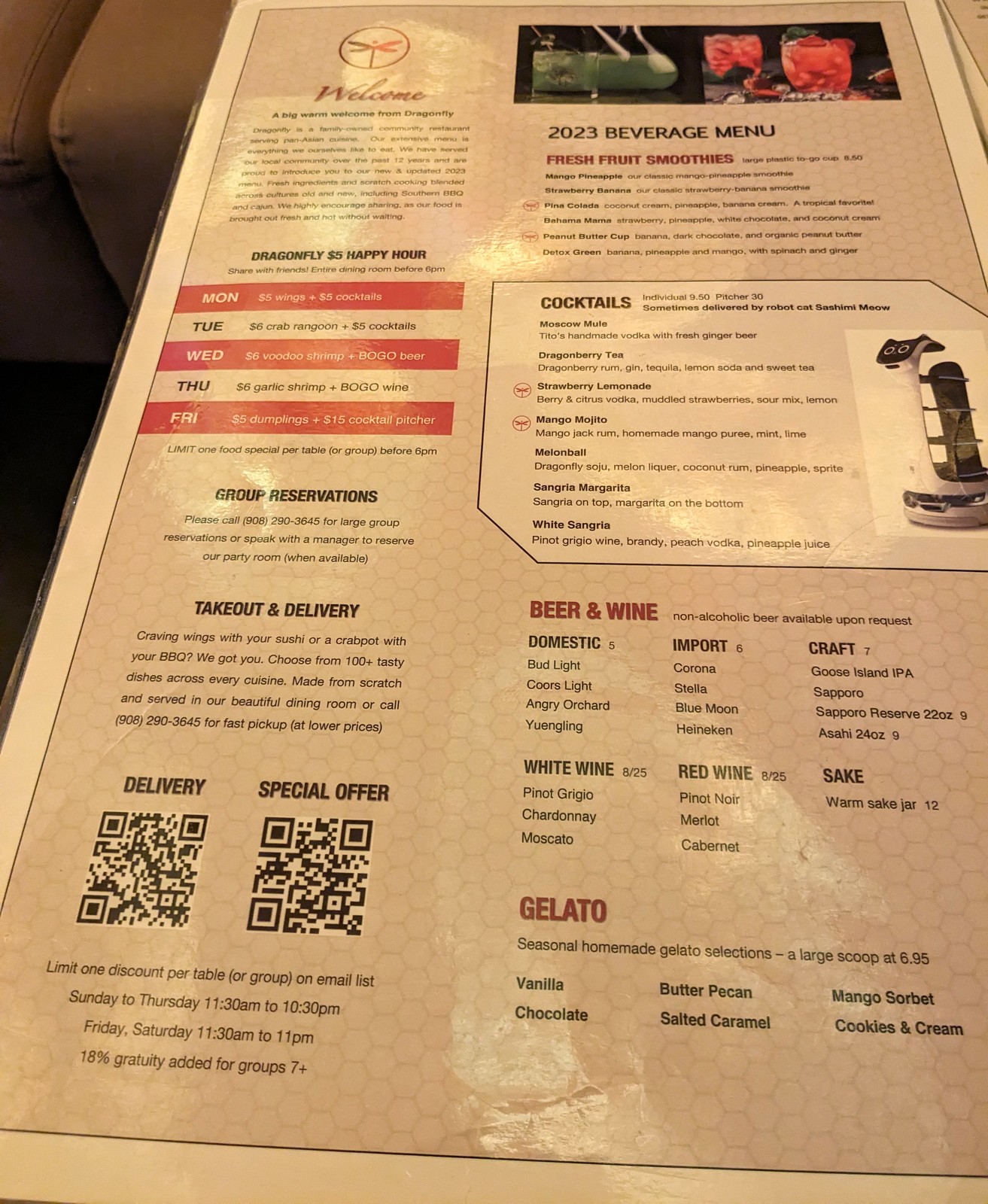A detailed menu image is depicted, primarily centered on the upper left-hand side. The most prominent feature is a menu with a cream-colored outer border and a very light reddish-brown interior. At the top, a circular logo features red wings on the right, brown wings on the left, and a small dot and line, with the word "Welcome" underneath in red. Below this, in small black text, unreadable due to the size, it states "Dragonfly $5 Happy Hour" followed by additional tiny black words.

The menu continues with distinct sections associated with each day of the week, highlighted by red rectangles with white text for "MON," "WED," and "FRI," and cream-colored sections with the black text "TUE" and "THU." Here, additional smaller, unreadable words are present.

Further down, in black text, it states "Group Reservations" followed by more tiny words. Another section labeled "Takeout and Delivery" appears, with yet more small text underneath. Below is the delivery information, encompassing a QR code followed by another section titled "Special Offer" with a QR code underneath. Text regarding limited discounts and operational hours spans across Sunday to Thursday from 11:30 a.m. to 10:30 p.m. and Friday to Saturday from 11:30 a.m. to 11 p.m., along with an 18% gratuity note for groups of seven or more.

On the upper right-hand side, there's a picture with indistinct green and tan elements on a blackish background, presumed to showcase cocktails. Underneath, in black text, it reads "2023 Beverage Menu," followed by "Fresh Fruit Smoothies" in red, with additional black text too small to decipher.

A more three-dimensional rectangular section titled "Cocktails" is present, with subsequent tiny unreadable writing and two small symbols at the top of the menu beside unspecified drinks. An unclear image of a white and gray machine appears. In red, it states "Beer and Wine" adjacent to further tiny, unreadable text.

The menu's domestic beer section includes Bud Light, Coors Light, Angry Orchard, and Yuengling. The imported beer section lists Corona, Stella, Blue Moon, and Heineken. The craft beer section includes Goose Island IPA, Sapporo, Sapporo Reserve (22 oz.), and Asahi (24 oz.).

In black text, the white wine section lists Pinot Grigio, Chardonnay, and Moscato, while the red wine section enumerates Pinot Noir, Merlot, and Cabernet. Additionally, it offers "Warm Sake Jar" under the Sake section.

Lastly, in red, it says "Gelato.” The seasonal homemade gelato selection is detailed in black, listing Vanilla, Chocolate, Sorbet, Butter Pecan, Salted Caramel, Mango Sorbet, and Cookies and Cream. Each large scoop is priced at $6.95.